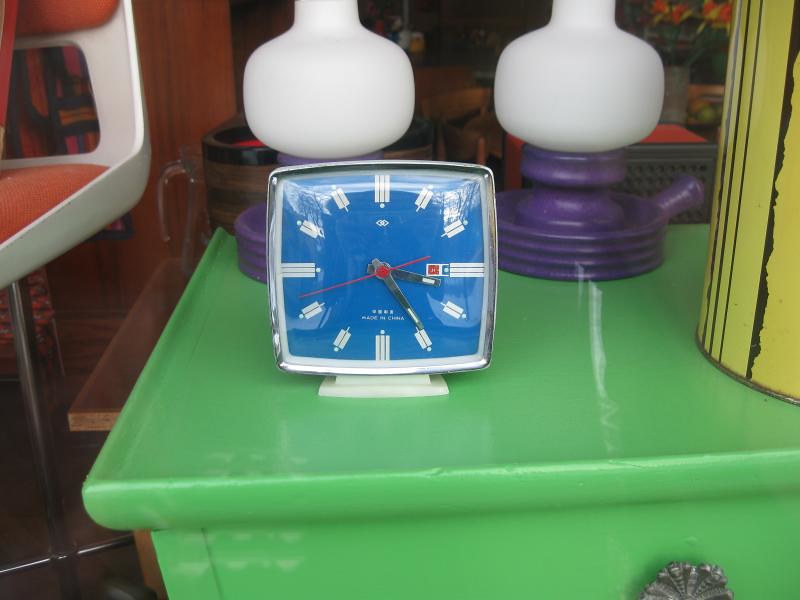This photograph, likely taken at an antique store or estate sale, showcases a fascinating mix of vintage and futuristic elements. The central focus is a sleek, modern-looking clock with a silver, square frame. The clock's face is a striking royal blue adorned with white, non-Roman numerals arranged in a unique pattern of columns: three columns at the center and then alternating sequences of two and three columns around the dial. The time is indicated by grayish-black hour and minute hands and a thin, red second hand.

The clock rests on a vibrant green table made from a material reminiscent of old Pyrex bowls. Flanking the clock are two peculiar lamps or lanterns with dark purple bases, which give off a whimsical, plunger-like appearance. These bases support white lantern tops, creating a striking contrast.

Towards the right side of the table, a yellow painted metal object, possibly the side of a trash can, adds another layer of intrigue. On the left, a retro 1960s-style stool catches the eye with its metal frame and bright orange cushioned seat set against a white base.

In the background, although somewhat indistinct, more assorted items hint at the eclectic array of treasures available in the store. This image beautifully captures a blend of mid-century modern, retro, and futuristic design elements, making it a captivating snapshot of a moment frozen in time.